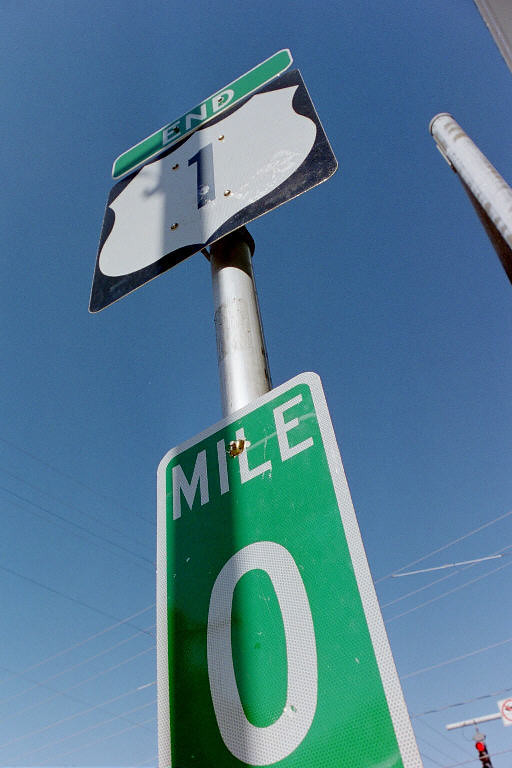This photograph captures a road sign from a low angle, as if the photographer was squatting to take the shot. The sign is mounted on a silver metal pole. There are two main parts to the sign: 

1. At the top, there is a green square with the word "END" written in white letters.
2. Below it, a rectangular green sign with white text displays "MILE" and "0", indicating mile zero.

Between these two, a white sheriff's badge-like emblem features the number "1" in black, symbolizing the end of Highway 1. The background showcases a beautiful, clear blue sky, enhancing the prominence of the sign.